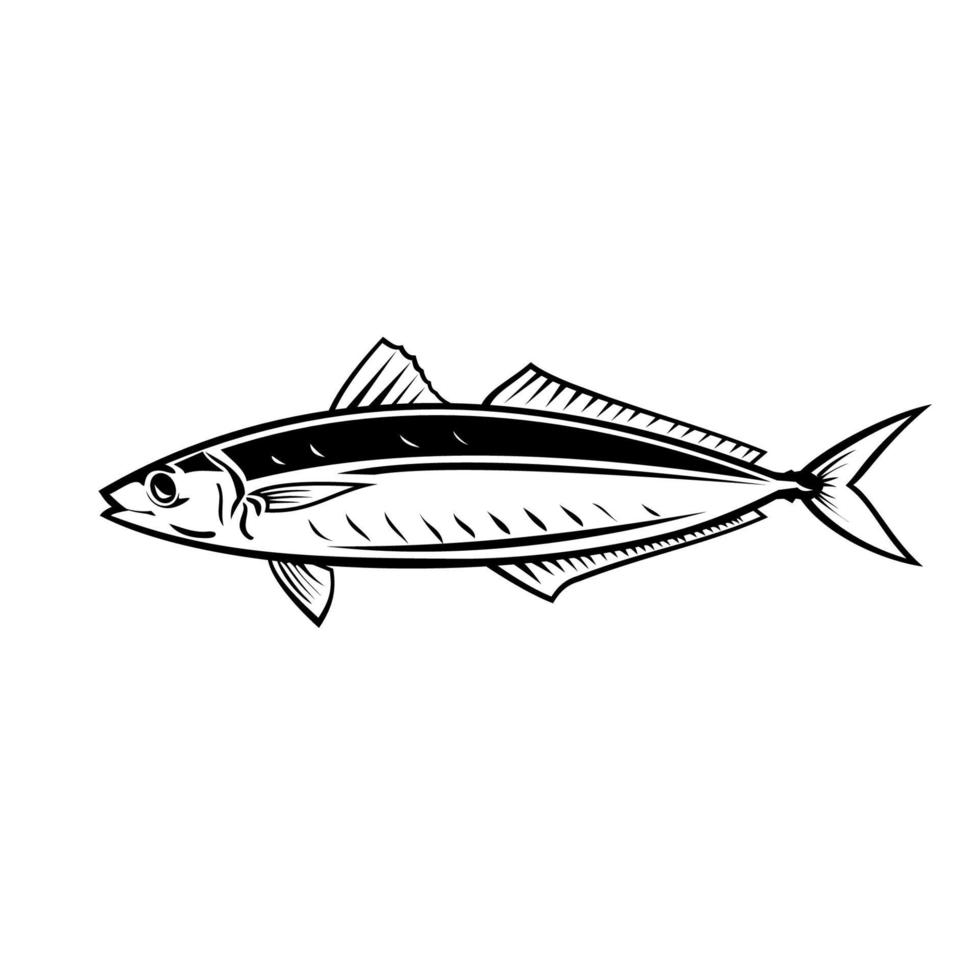This image is a detailed black and white drawing of a long, slender fish, facing left. The drawing is simple yet intricate, with clean lines and shading that suggest a shadow effect, giving the fish depth and dimension. It displays five fins: two elongated ones on the top, two on the bottom, and one on the side. The tail is standard with a two-pronged shape. The fish features detailed gills and an eye highlighted with a white streak, which makes it appear somewhat lively. The overall style resembles an old-fashioned diagram, possibly used for identifying specific fish species, such as in books or informational signage about permissible catches. The stripe above its body and the use of thick black outlines add to its definition, making it clear this is not a generic fish but a specific kind, potentially useful for educational or illustrative purposes.